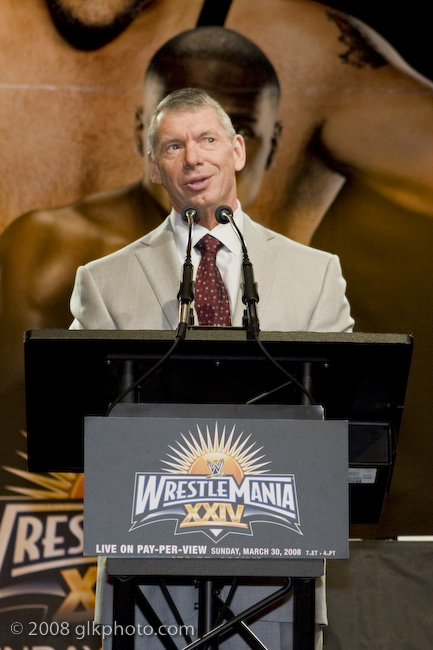The photograph captures a man standing behind a black podium adorned with a black card reading "WrestleMania XXIV" and white text stating "Live on Pay-Per-View, Sunday, March 30, 2008, 7 Eastern, 4 Pacific Time." The podium, slightly sloped towards the man, features two black microphone stands aimed at him. He is dressed in a tan suit jacket and pants, a white button-up collared shirt, and a red tie with gray dots. His mouth is open in a smile, and he is looking towards the right with his head tilted slightly to the left. The man has short, graying hair with hints of brown. At the very bottom left corner of the photograph, white text overlay reads "Copyright 2008 glkphoto.com." The background features indistinct figures, including a black man and another individual, but they are not clearly visible.